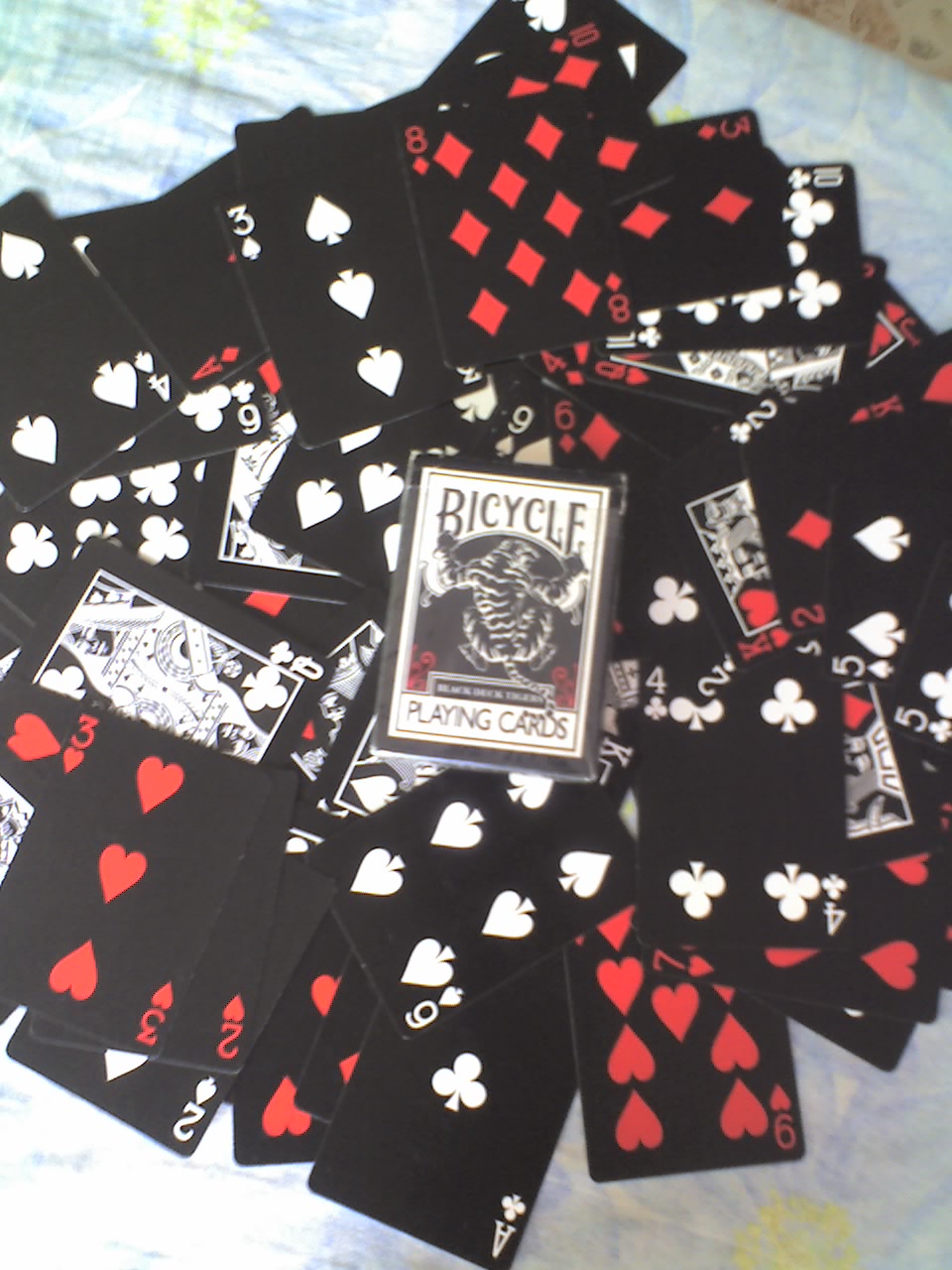Close-up of a circular arrangement of playing cards on a silvery gray, textured surface. The focal point of the image is a box of playing cards positioned prominently at the center of the pile. The box features a design in red, black, and white hues, with "Bicycle Playing Cards" written in bold black text on its surface. Surrounding the box, the visible cards showcase various faces: a black background with a six of spades, three of spades, eight of diamonds, three of hearts, nine of hearts, and three of diamonds. The stack is abundant, hinting at many more unseen cards beneath the top layer.